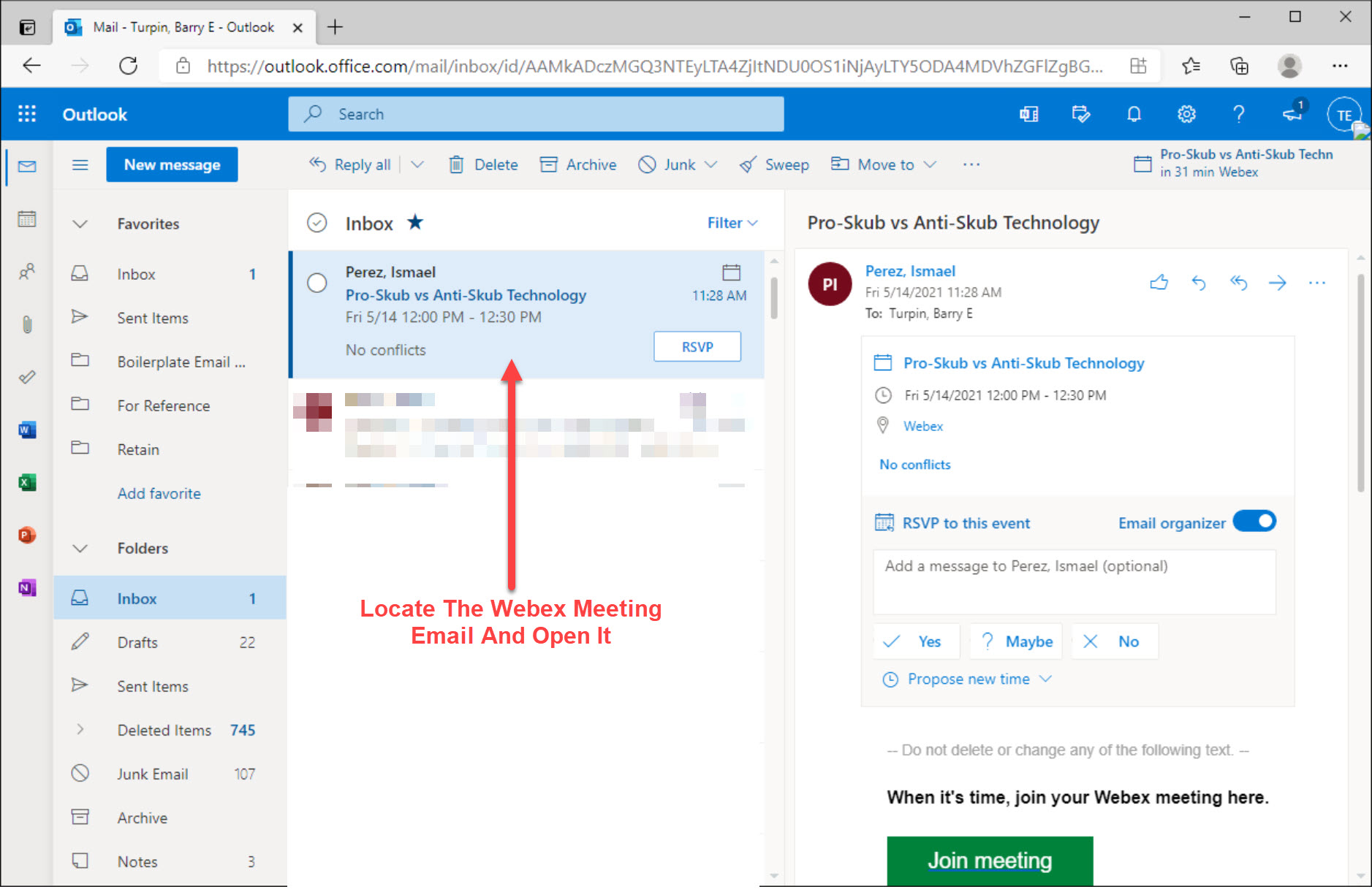The image depicts the email interface of a website, likely Microsoft Outlook. In the upper left-hand corner, there is a light gray banner featuring an icon on the far left, followed by an open tab labeled as "Mail," indicated by an email symbol next to the text "Tuppenberry E Outlook."

Directly below this banner, there is a navigational bar containing a back arrow, a forward arrow, a refresh arrow, and an address bar with the URL beginning with "HTTPS" accompanied by a lock icon. To the right of the address bar, there are three icons outside of the search field.

Further down, a blue banner stretches across the screen. On the far left of this banner is a square icon divided into nine smaller squares, indicative of an app launcher. "Outlook" is written next to this square, followed by a sky blue search area. Towards the right of the banner, there are several icons including a bell (likely a notifications icon), another application icon for Microsoft, and a circular profile icon.

On the left side of the screen, flush with the edge, are additional icons. Prominently displayed in the middle of the screen is a long red arrow pointing towards an email related to a WebEx meeting, instructing the viewer to open it. To the right, there is content concerning "pro vs. anti-scub technology," providing details about a meeting along with a green "Join Meeting" button.